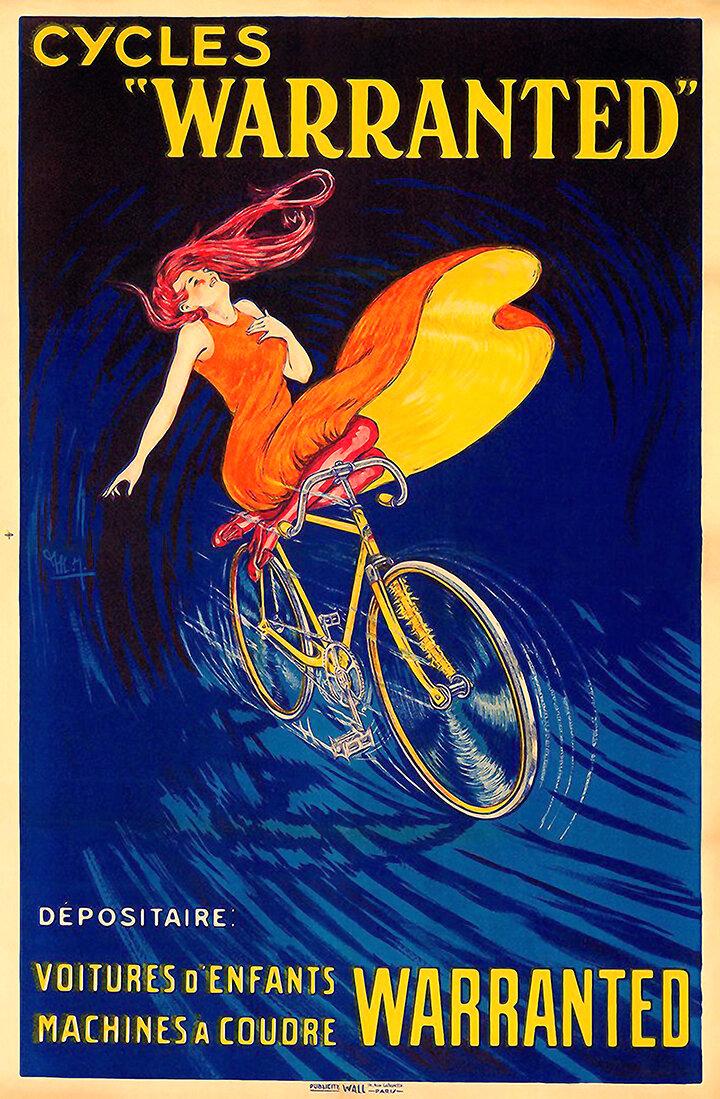The poster, with a tan border, prominently features a vibrant and dynamic illustration set against a swirling black and blue background. At the top, in bold yellow letters, it reads “Cycles ‘Warranted’.” The main focal point is a woman with flowing red hair, dressed in an orange dress with yellow accents, red stockings, and red shoes. She is seated sidesaddle on a yellow bicycle, her left hand clasped over her chest while her right arm extends outward. Her head is thrown back, exuding an air of carefree joy as her hair flutters in the wind. The bicycle is depicted with motion lines on the white and gray wheels, suggesting it is speeding towards the right. The lower part of the poster features white and yellow French text: “Dépotsitaire: Voitures d’Enfants, Machines à Coudre,” with the word "Warranted" repeated. The whole composition is intricately hand-drawn, encapsulated by a light yellow outline.